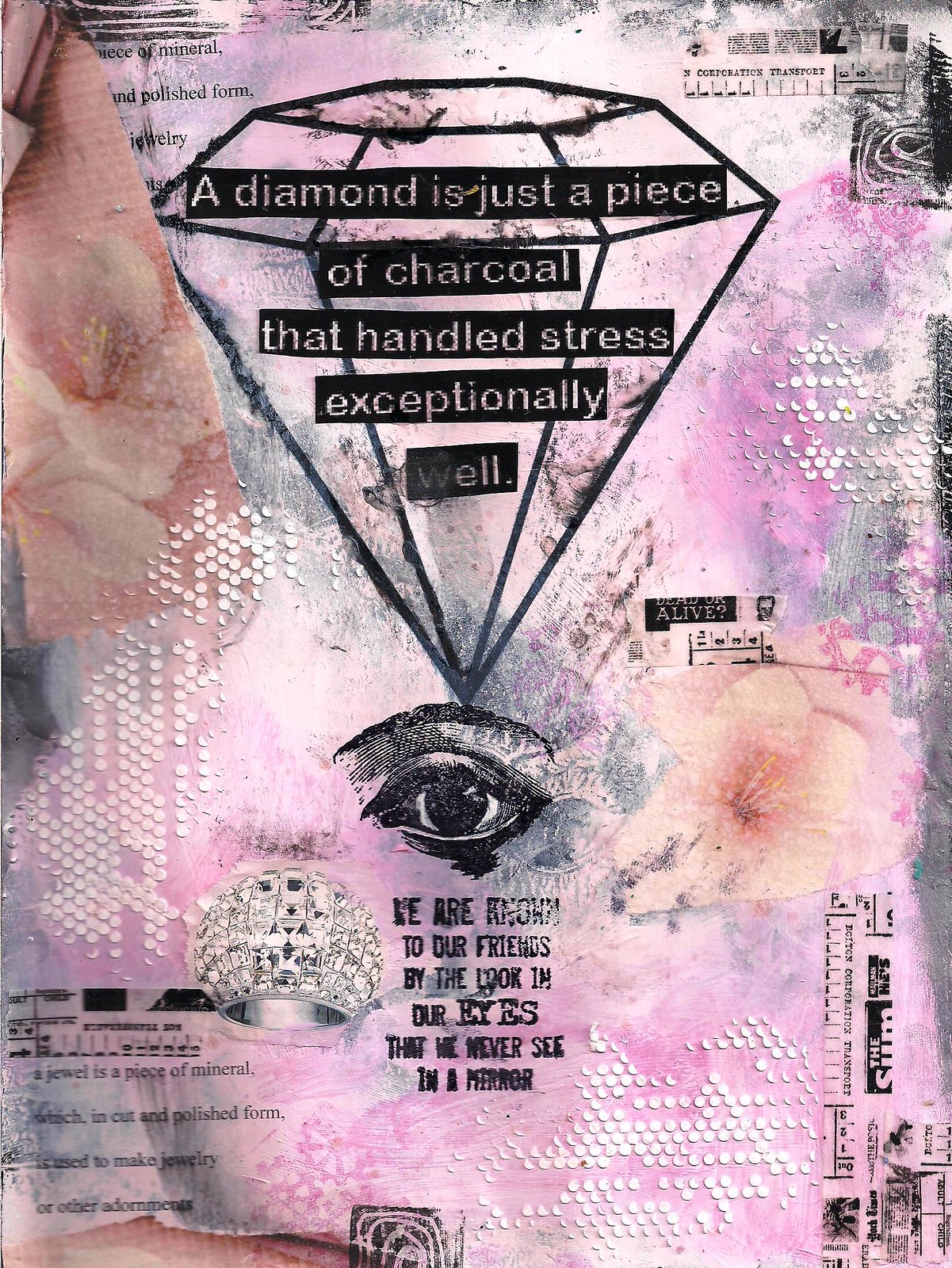This vertically-oriented art collage features a distressed, molted-style background splattered with shades of pink, gray, silver, and subtle touches of light purples. The textured backdrop, reminiscent of a chalk explosion, creates a smeary, blotched effect over which various elements are arranged. Dominating the upper section of the image, a large line art drawing of a diamond sits centrally, its geometric shape widening at the top and tapering to a sharp point at the bottom. Overlaid on the diamond are black bars with white text, reading: "A diamond is just a piece of charcoal that handled stress exceptionally well."

Beneath the diamond illustration is a meticulously detailed, lithograph-style drawing of a wide-open human eye, adorned with an arched eyebrow and heavy, dark lashes. Below the eye, in black text that is challenging to read against the distressed background, is the phrase: "We are renowned to our friends by the look in our eyes that we never see in a mirror."

Scattered across the collage are additional elements, including a light pink flower near the right-center, a diamond-studded ring to the left, and areas of unclear black markings and text that add to the overall textured aesthetic. The image employs a vibrant palette of pinks, grays, blacks, whites, peach, and purples, contributing to its hyper-stylized and richly layered appearance.